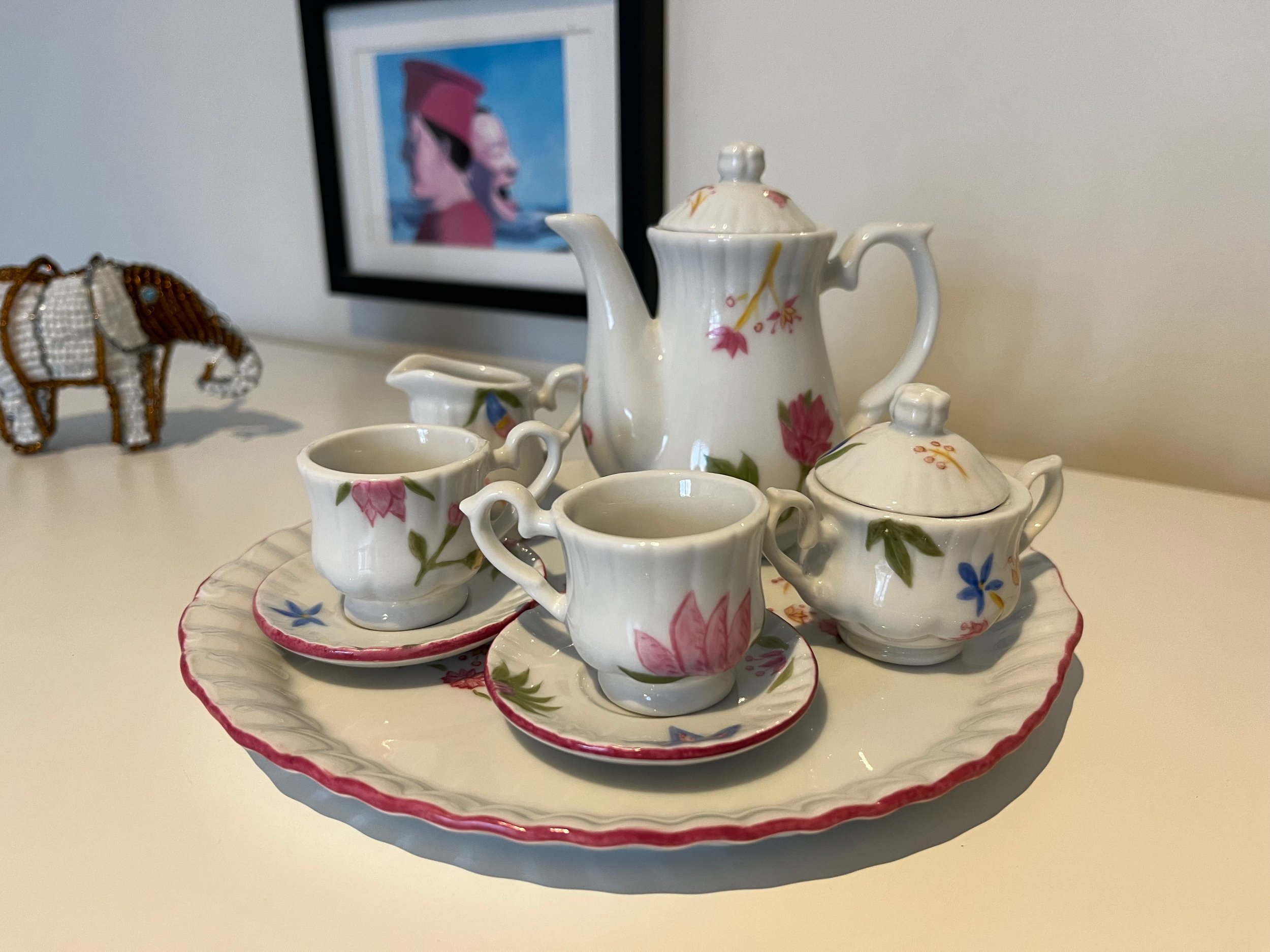In this detailed and quaint scene, a delicate ceramic tea set graces a white tabletop. The tea set, possibly miniature, includes a ruffled, fluted serving plate with white and pink trim, mirroring the elegance of a bygone era. Central to the ensemble is a teapot surrounded by a sugar bowl, a creamer, and two coffee cups, each resting on its saucer. The tea set is richly adorned with a floral design that features pink and blue flowers interwoven with green leaves, set against a pristine white background.

To the left of the tea set, a small beaded elephant made with brown and white beads adds a touch of handcrafted charm, facing towards the right. In the background, hanging on a white wall, is an intriguing painting within a black frame and a white mat. The artwork depicts a dual-faced person: one face solemnly staring left, while the other face, emerging from the back, is expressive, perhaps laughing or screaming, providing a thought-provoking contrast.